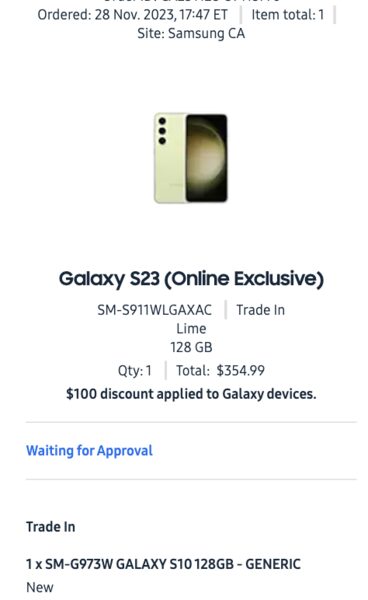In the photograph, captured from a mobile phone, you are given a glimpse into the process of trading in a Samsung Galaxy S23. The top portion of the image is slightly cut off but clearly states "Ordered 28 November 2023" at 17:47 ET. The site listed is "Samsung CA." The item details show a quantity of one, with a thumbnail image of the phone.

The phone's front appears shiny, and the back features three cameras, indicative of modern smartphone designs. There is also a glowing moon-like icon visible on the screen. The text "Galaxy S23 (Online Exclusive)" is clearly noted, alongside the model number "SM-5911WLGAXAC." The trade-in color is specified as "Lime," with a storage capacity of 128GB, quantity one. The total cost listed is $354.99, annotated with a "$100 discount applied to Galaxy devices." 

The current status says "Waiting for Approval" in blue text. Further down, the phone details list it as "Generic," with a condition noted as "New" in black print. This detailed glimpse provides insight into the trade-in process, showcasing the order specifics and the significant details involved.